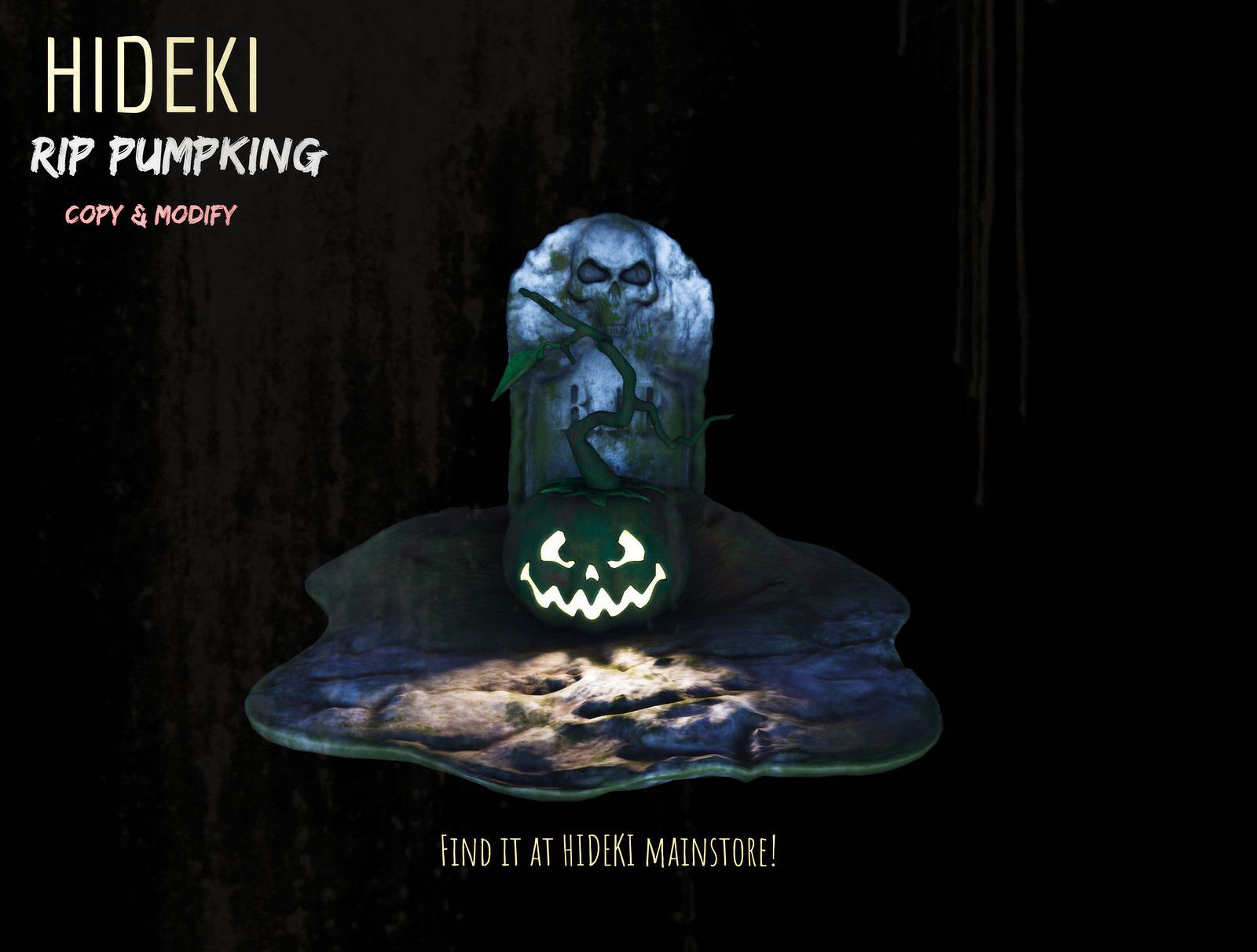The image is a 3D render set in a floating, gray gravel-like ground within a black void. Dominating the scene is a glowing green jack-o-lantern with a large stem sprouting leaves. Beside it stands a detailed gravestone, inscribed with "Rest in Peace" and topped with a skull featuring large black eyes. Blood-like, gray splatters and drips decorate the black background. In the top left corner, large yellow text reads "Hideki," followed by bold white text stating "R.I.P. Pumpkin." Below this, in small orange letters, it says "Copy and Modify." At the bottom of the image, yellow text declares, "Find it at the Hideki Main Store," suggesting a Halloween-themed promotional piece. The light from the jack-o-lantern reflects eerily on the ground, enhancing the spooky atmosphere.